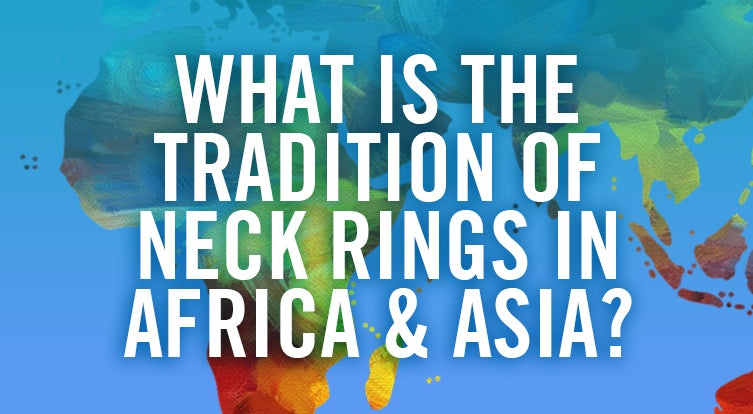This image features a vibrant and detailed depiction most likely intended for a PowerPoint presentation. Dominating the center of the picture in large, bold, white capital letters is a question: "What is the tradition of neck rings in Africa and Asia?" This text is spread across four lines and stands out starkly against the visually engaging background.

The background itself is an artistic and abstract representation of the maps of Africa and the lower half of Asia. The image utilizes an ombré spectrum starting with various shades of blue and teal at the top, transitioning into greens, pale yellows, and culminating in striking oranges, browns, and reds towards the bottom left. The colors suggest a watercolor or painted aesthetic, reminiscent of the illustrative style of Eric Carle, with a textured, collage-like appearance.

At first glance, the background appears to be an oceanic scene with its predominant blue tones. However, upon closer inspection, the shapes and shifting colors reveal the continents. The overall impression is one of a highly colorized and abstract map that not only captures attention but also adds a level of intrigue and depth to the image's central textual question. The details in the background become progressively clearer from the top to the bottom, adding to the dynamic visual appeal of the image.